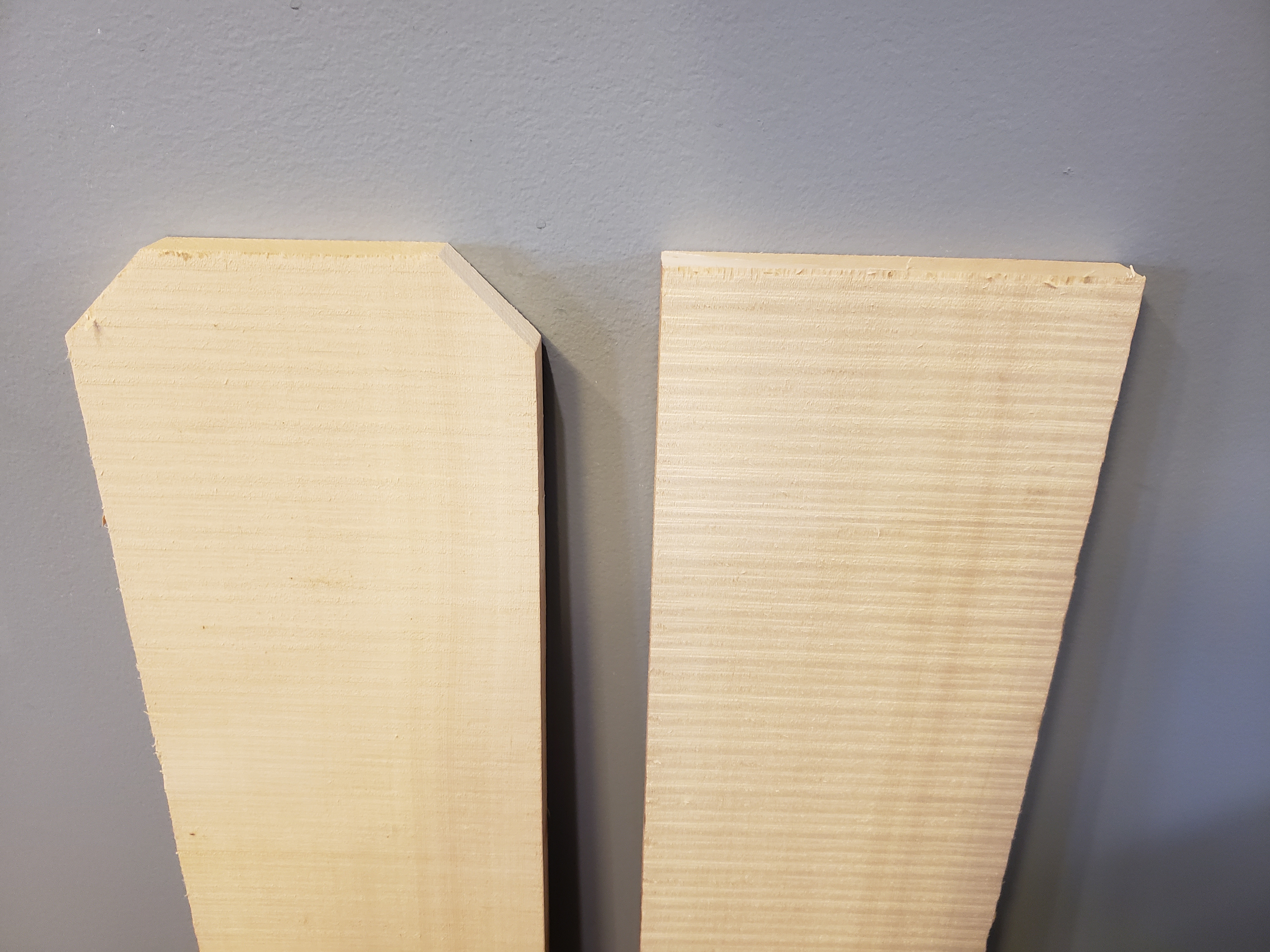The image presents two distinct wooden planks leaning upright against a white plaster wall. The wall itself is stark and textured with typical plaster finishes. The first plank is straightforwardly rectangular in shape, showcasing typical grain patterns and edges. In contrast, the second plank features a more complex geometry – it’s hexagonal with its left and right sides being the longest parts. These sides gradually taper off at the ends, forming angled cuts that appear to create a secondary, smaller flat section at each terminus. The wood of the hexagonal plank is gray-toned, possibly indicating a type of weathered or aged wood. Both planks exhibit rough, visibly unfinished edges and the top ends particularly highlight this unfinished quality, suggesting recent manual cuts rather than machine precision. This roughness gives the impression that the planks might have been hand-crafted or altered at home rather than being store-bought in their current state.